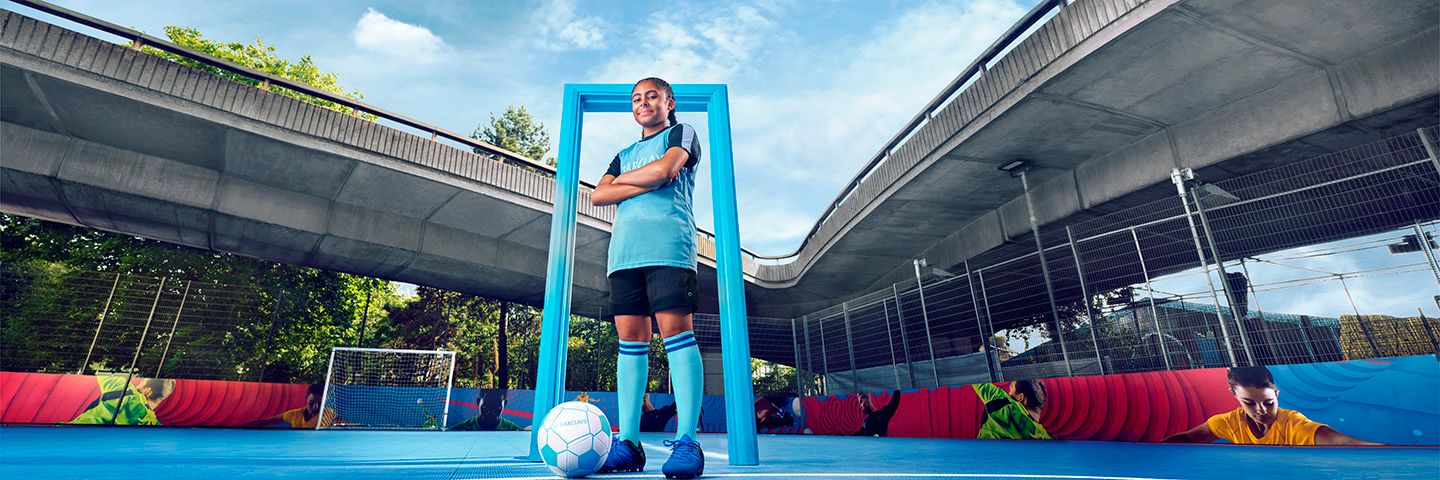This panoramic wide-angle photograph captures a vibrant scene outside under a bright, sunny sky. Central to the image is a young teenage girl, possibly a soccer player, standing confidently with her arms crossed. Dressed in a light blue jersey with darker blue accents on the cuffs, dark blue shorts, and blue knee-high socks featuring dark blue bands at the top, she completes her ensemble with bright blue sneakers. In front of her, a soccer ball rests on a blue-colored surface that matches her outfit. 

The setting appears to be an adaptive reuse urban park situated beneath intersecting concrete bridges that converge at a point in the background. Behind her, a light blue door frame adds a contrasting structure, and to one side, a freestanding soccer goal is visible. Along the bottom of an enclosed chain-link fence, a mural depicting children engaged in various sports stretches across, adding a lively element to the scene. This detailed composition showcases the girl's strong presence amidst a dynamic and colorful urban sports environment.